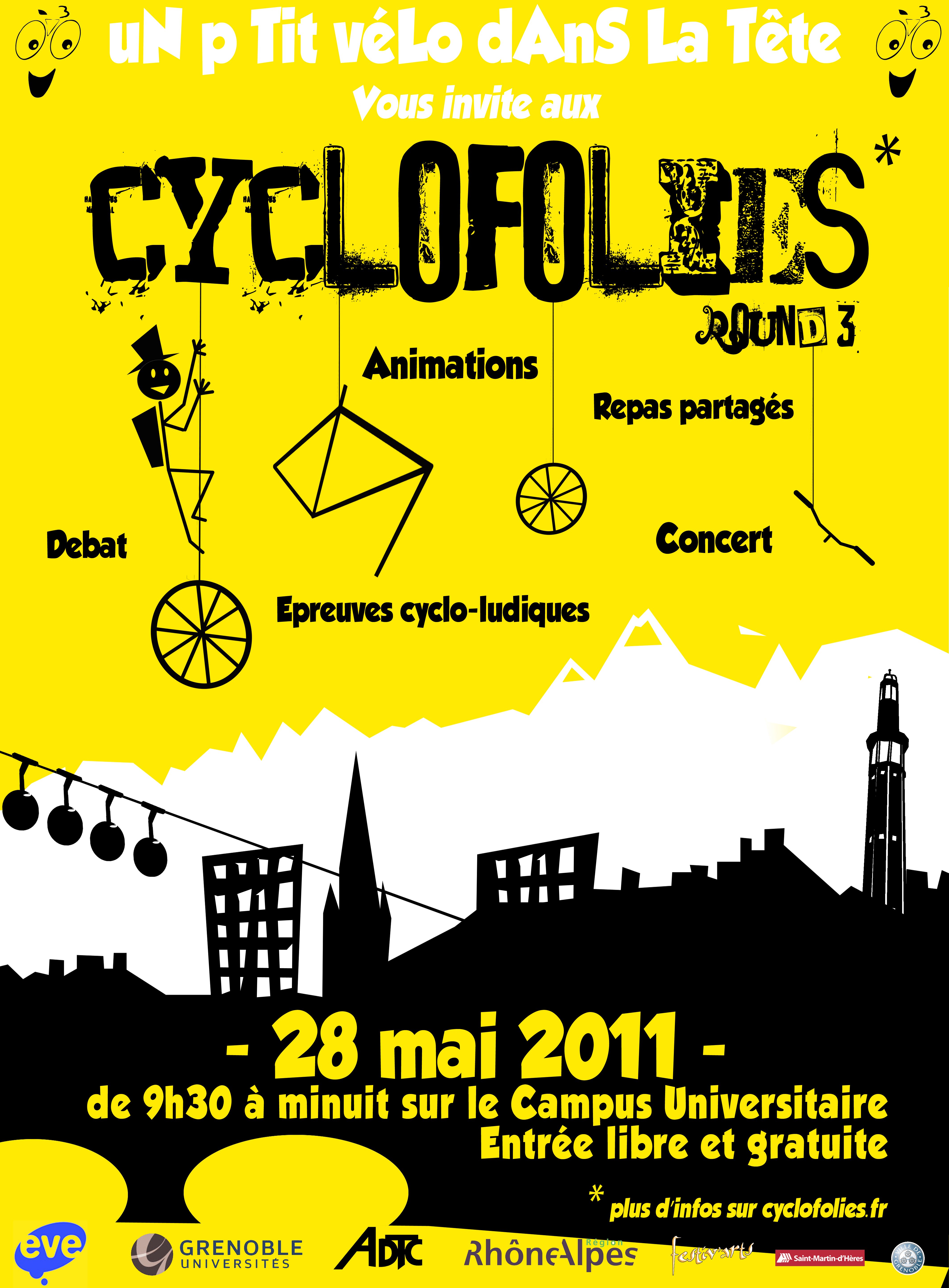This vibrant and intricately designed poster promotes an event called "Cycle Follies" (Cyclofolies), scheduled to take place on May 28, 2011, from 9:30 AM to midnight at a university campus, likely the Cerro de la Campes Universite. Dominated by a yellow background, the top region of the poster features corner smiley faces with bicycle wheels for eyes. The bold title "Cyclophiles" is accompanied by an asterisk and whimsical illustrations – including a man climbing a unicycle while wearing a backpack and top hat, plus dangling bike parts like wheels and handlebars. Key event highlights such as "Animations", "Concert", "Round Three", "Debat", and "Cyclodasludiques" are prominently listed. A white outline of mountains separates the yellow upper portion from a black cityscape below, which includes a gondola wire. The lower section of the poster displays the event date and time, along with logos of various sponsors: Eve, Grenoble Universities, ADTC, and Roan Alps, with three other illegible logos. The poster is in French, adding to its eclectic and engaging visual appeal.